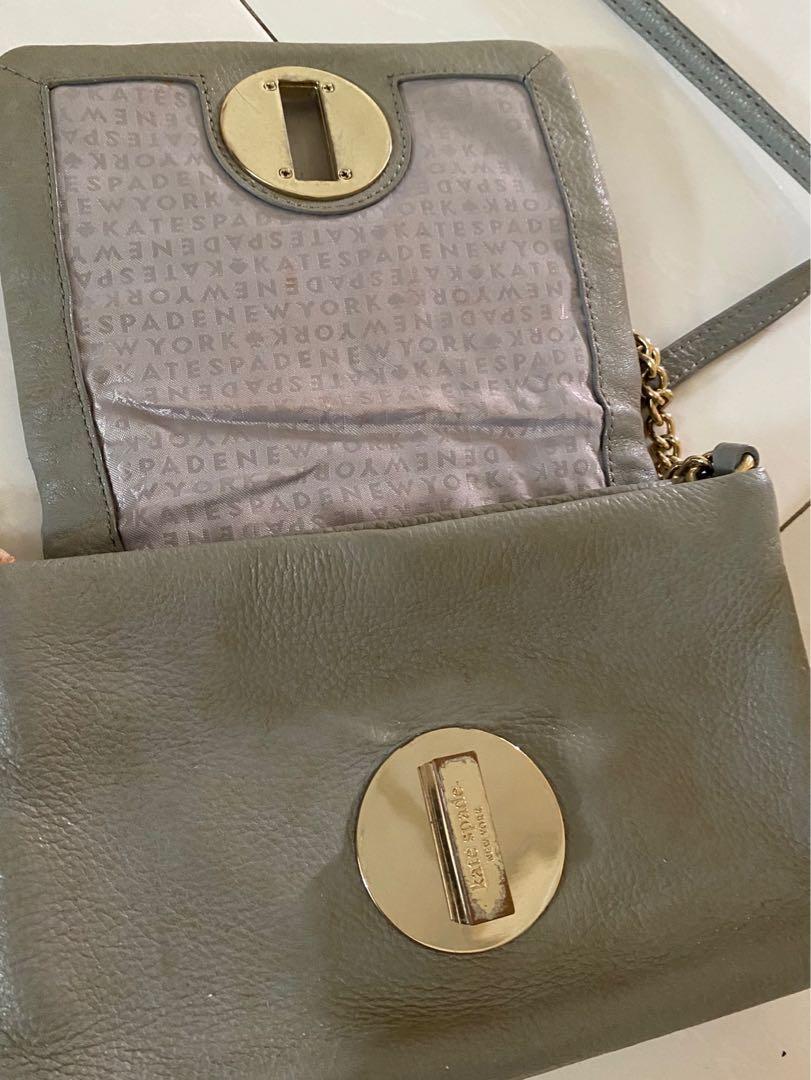An image features a well-loved handbag from the brand Kate Spade New York. The handbag is dark gray with a noticeable gold clasp at its center, though the clasp appears significantly worn. A hint of a gold chain suggests it can be draped over the shoulder, while a dark gray handle offers an alternative carrying option. The handbag is open, revealing an interior lined with fabric pattern adorned with the Kate Spade New York logo. The wear on the edges and clasp is evident, showcasing its extended use. The handbag is set against a plain white tiled floor, which does not provide a visual reference for the size of the bag.